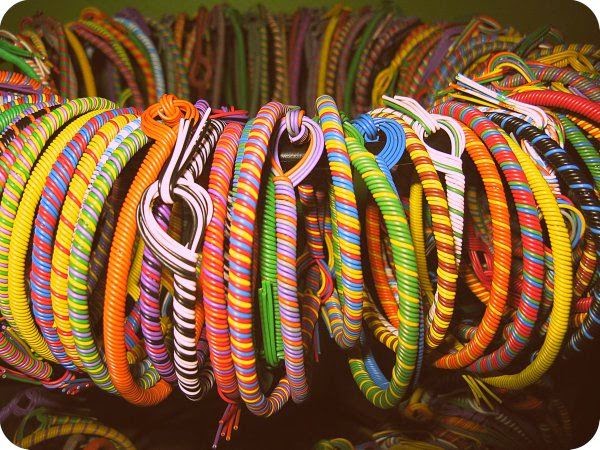The image showcases a close-up view of an extensive collection of meticulously hand-made bracelets, crafted from multicolored plastic threads. Each bracelet is brilliantly vibrant, featuring a variety of colors including green, yellow, red, pink, purple, black, white, blue, gold, cyan, orange, and more. The bracelets are predominantly multicolored, with many displaying alternating candy-cane stripe patterns, while some are solid in color.

All bracelets share a uniform knotting technique and are uniformly tied, displayed on what seems to be a round black structure that allows them to hang neatly in a circular arrangement. The image focuses solely on these bracelets, ensuring they are the central feature. The bright and clear setting, coupled with the vivid and striking color contrasts, highlights the craftsmanship and variety of these plastic thread bracelets, making them appear both well-made and eye-catching.